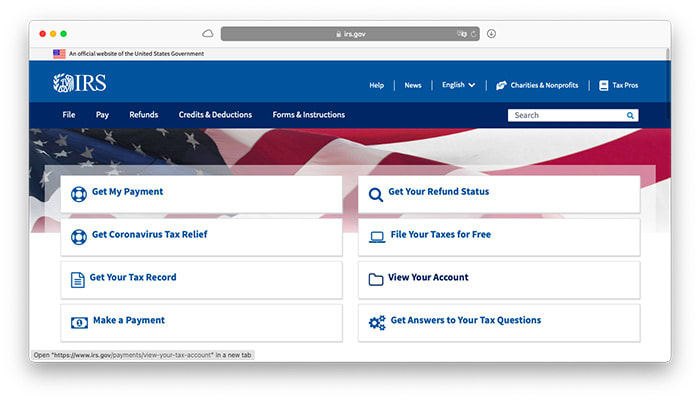This is a detailed screenshot of the IRS website. The URL bar at the top of the page is dark gray with white text, displaying "IRS.gov." Just below the URL bar, the title of the webpage appears in the upper-left corner, accompanied by a small American flag and the text "An official website of the United States government."

The main portion of the website starts just beneath this section, featuring a blue background. In the top-left corner of this area, the IRS logo is prominently displayed next to the letters "IRS." To the right of the logo is the site’s navigation menu, which includes several buttons: "Help," "News," and a language selector set to English. Adjacent to these buttons are links labeled "Charities & Nonprofits" and "Tax Pros," which likely offer information and resources for charitable organizations and tax professionals, respectively.

In the main body of the webpage, multiple selection buttons are available for various services:
- "Get My Payment"
- "Get Your Refund Status"
- "Get Your Coronavirus Tax Relief"
- "File Your Taxes for Free"
- "View Your Account"
- "Get Answers to Your Tax Questions"
- "Make a Payment"
- "Get Your Tax Record"

The background in the central part of the website prominently features the American flag.